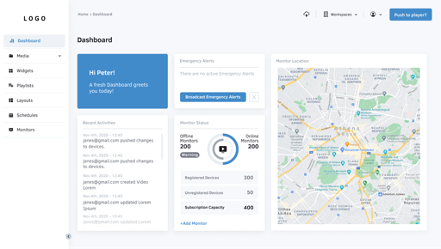The image depicts a screenshot of a website viewed from a distance, with certain details being discernible. In the top left corner, there is a bold, black font heading which appears to say "Logo". Directly beneath this heading, there is a highlighted word in grey with text in blue font, though the exact wording is unclear. The navigation menu contains six additional selections, each situated beneath the highlighted item.

The main content is titled "Dashboard" and is organized into three columns. The first column features a blue box displaying the greeting "Hi Peter", accompanied by some text below it. Beneath this, there is another box aligned to the left, containing various bits of information.

The middle column includes a small box on top and another box below, the latter having an icon resembling a play button encircled by a partially blue ring.

The right column showcases a map, likely representing some type of community layout or regional area. The overall layout and structure suggest an organized dashboard interface with multiple interactive elements.